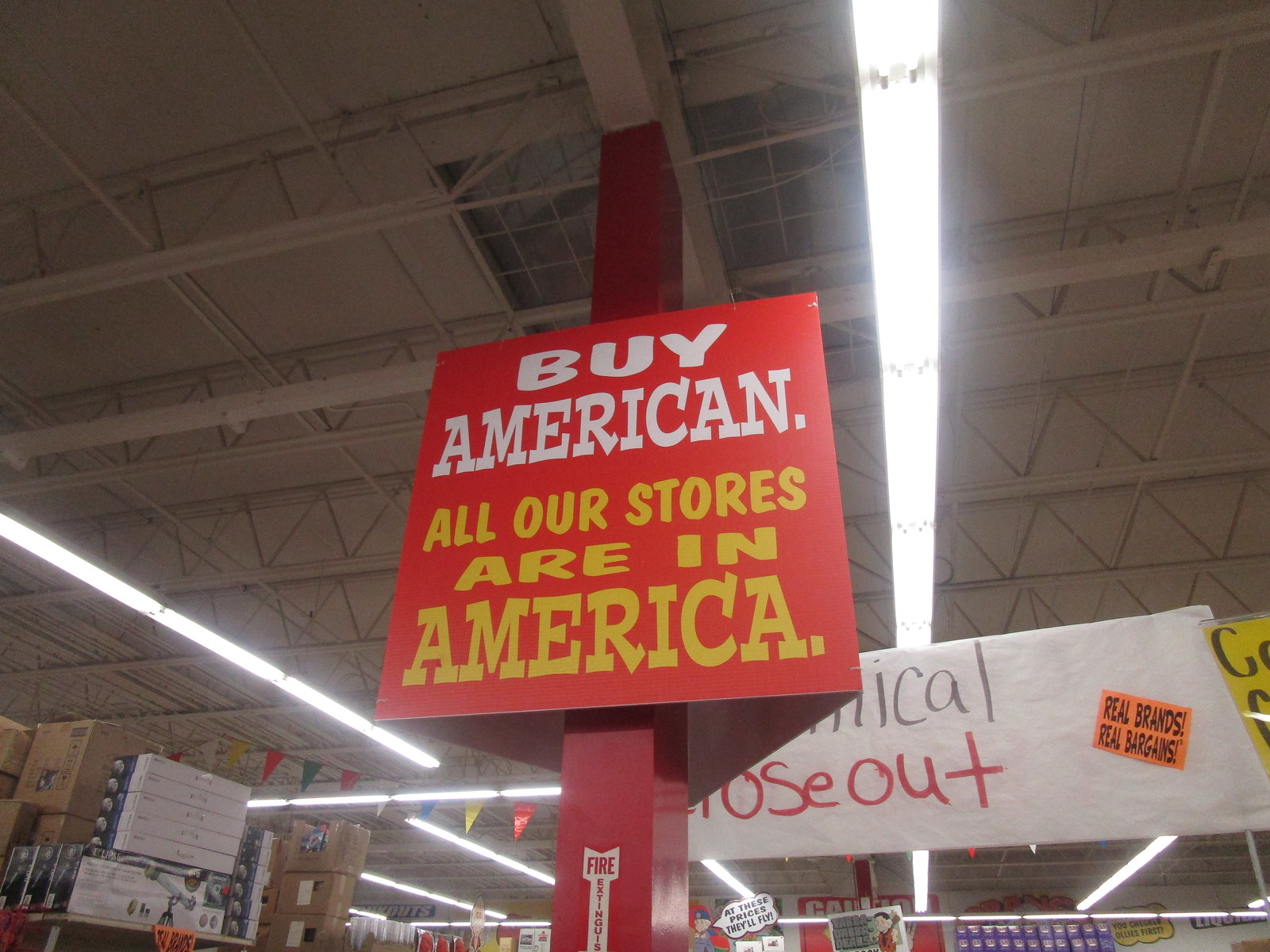The image depicts an interior view of a large warehouse store. Dominating the foreground, a prominently positioned red square sign hangs from a central red post. The sign bears the message "Buy American" in bold white font, followed by "All our stores are in America" in striking yellow letters. Below this main sign, there is a smaller white sign displaying the partially obscured text "Close Out" in vivid red letters, accompanied by an orange sticker that reads "Real Brands, Real Bargains." The store’s airy ceiling features vast beige rafters interspersed with long, slender hanging lights, extending out of view and illuminating the expansive space. In the background, rows upon rows of shelves are stacked with a variety of brown and white boxes, creating a sense of depth and abundance. Scattered banners add to the visual complexity, reinforcing the vibrant, bustling warehouse environment.